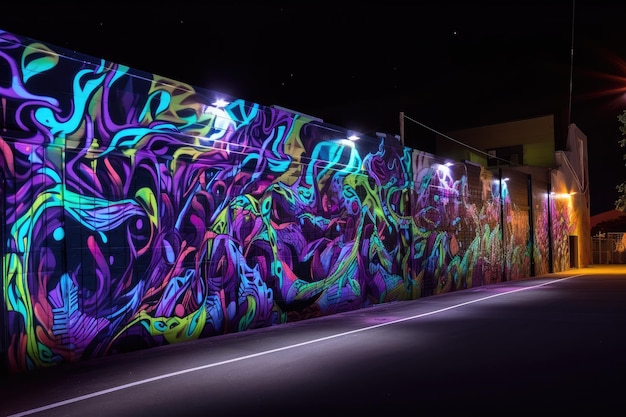The image depicts a vibrant, large-scale graffiti mural adorning the side of a two-story brown building in an urban setting, captured at night. The mural, which spans the entire length of the building from the far side to a doorway, features dynamic purple and blue swirls complemented by neon green, yellow, pink, and white highlights that create a striking, futuristic aesthetic. The colors are illuminated and intensified by black lighting, making them glow vividly against the dark night sky. In the foreground, a sidewalk and a street run parallel to the mural, with a long strip of black light casting a continuous luminescent glow on the artwork. The night sky above is deep black with a few scattered stars, adding to the overall nocturnal ambiance of the scene.